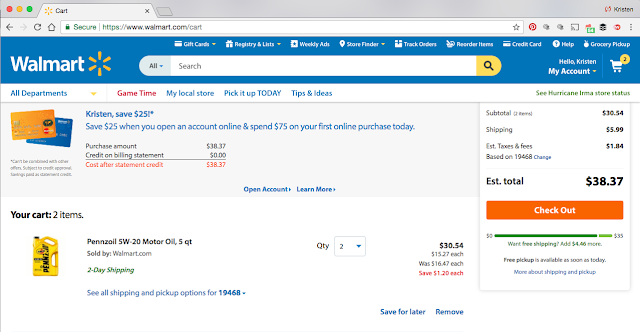A screenshot of a shopping cart on Walmart.com, as viewed on what appears to be an Apple computer based on the layout and design. The browser tab reads "Cart" next to the Walmart logo, and the URL shown is https://www.walmart.com/cart. The top banner features Walmart's signature blue color with the Walmart name and logo on the left.

At the top of the page, there are options for "Gift Cards," "Registry & Lists," "Weekly Ad," "Store Finder," "Track Orders," "Reorder Items," "Credit Card," "Help," and "Grocery Pickup." Below, there is a search box with dropdown options for specific categories and a search button. On the right side, it says "Hello, Kristin," indicating the account holder, with a link to "My Account." Next to this is a shopping cart icon with the number 2 in a yellow circle.

The white navigation bar includes options for "All Departments," "Game Time" in red, "My Local Store," "Pick It Up Today," "Tips & Ideas," and "See Hurricane Irma Store Status" on the far right. Below, there's an advertisement promoting a Walmart credit card offer, saying "Kristin, Save $25. Save $25 when you open an account online and spend $75 on your first online purchase today."

The shopping cart contains one item, a 5-quart container of 5W20 motor oil, with a quantity of two. The item is displayed with an image and its name. It is sold by Walmart.com with 2-day shipping indicated in green font. Shipping and pickup options are available for the zip code 19468. The extended description shows the quantity of two, costing $30.54 in total.

To the right, a box displays the subtotal, shipping costs, estimated taxes and fees, culminating in an estimated total of $38.37. Below this, an orange "Checkout" button is present. Additionally, there is a progress meter showing how much more needs to be added for free shipping, accompanied by a note on free pickup availability and a link to learn more about shipping and pickup options.